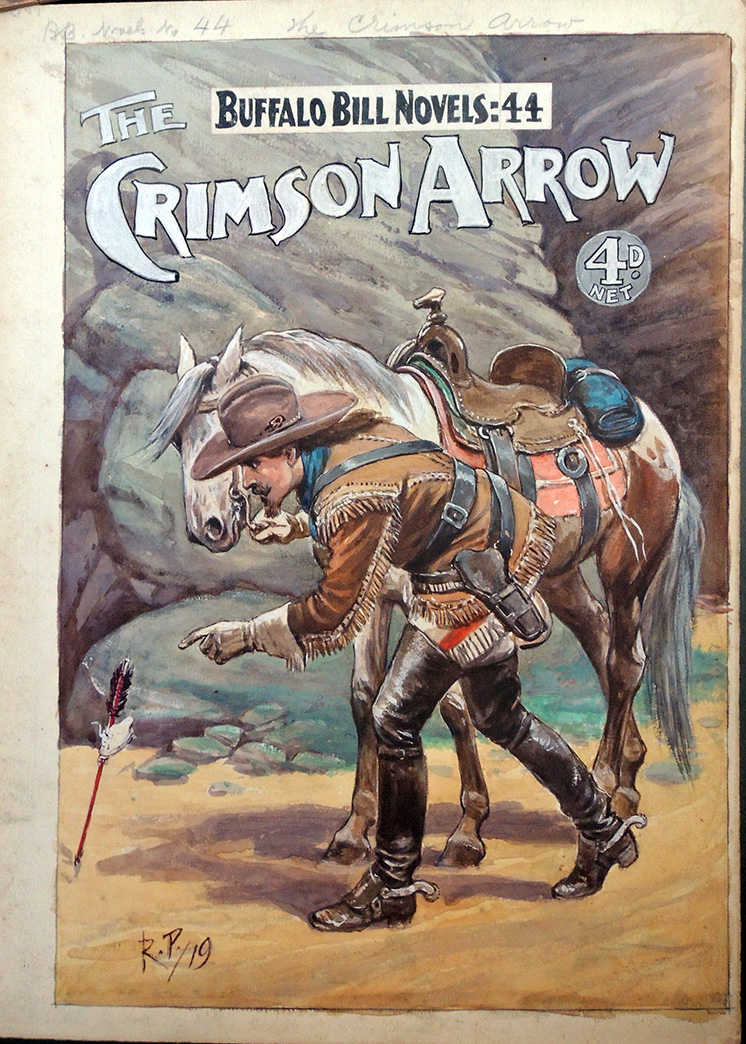The image, which resembles a painted picture from an old-school Wild West comic or a cover for one of the Buffalo Bill novels, depicts a vivid Western scene. At the top, within a rectangular white border with black lettering, it declares "Buffalo Bill Novels: 44." Below this, in gray contemporary modern writing, the title "The Crimson Arrow" appears. Additionally, there's a gray circle inscribed with "4D net" beneath the title.

The focal point of the picture shows a cowboy leading his white horse by the reins, rather than riding it. The horse, adorned with a brown saddle, a red saddle cloth, and a blue rolled-up sleeping bag behind the saddle, has distinctive brown markings on its back legs, a gray tail, and a blue blanket. The cowboy, dressed in a fringed, brown leather jacket with white leather gloves, black leather chaps, and knee-high black boots with spurs, also wears a brown hat. His attire is complemented by leather pants and a holster for his pistol.

In the scene, the cowboy is intently pointing to a feathered arrow shot into the ground, as if about to retrieve it. They are depicted walking on dirt, surrounded by towering cliffs and rocks that dominate the background, making it appear as though they are navigating through a canyon. Overall, the image captures a moment of suspense and discovery in a rugged, natural landscape, characteristic of early 1940s to early 1950s Western designs.